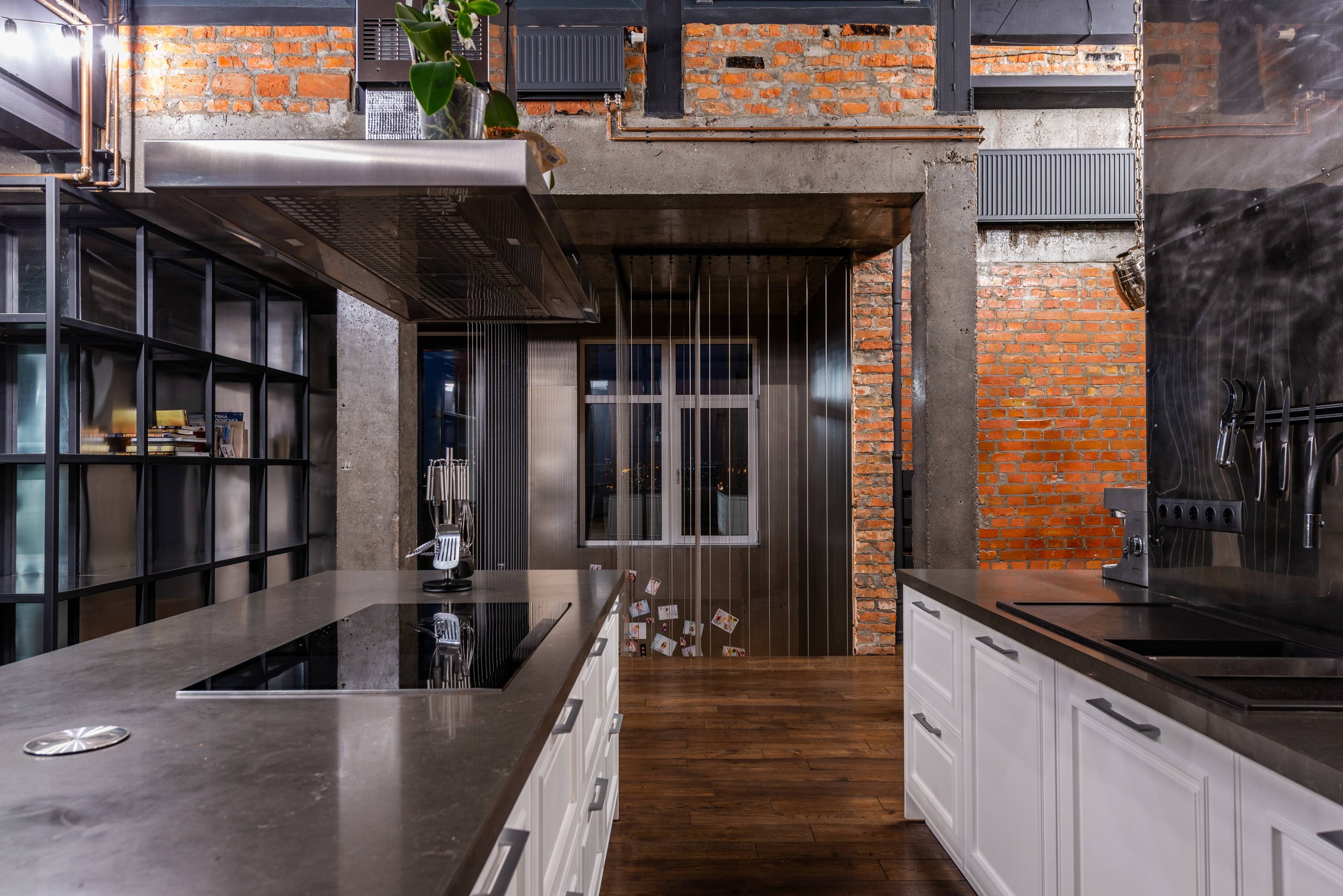This image features a sleek and contemporary kitchen with a distinct industrial and utilitarian aesthetic, set within what appears to be a loft or renovated warehouse. Dominating the backdrop are striking red brick walls and visible steel beams that contribute to its raw, industrial ambiance. The spacious kitchen boasts glossy, gray countertops, possibly made of sealed or glazed concrete, and features extensive counter space punctuated by a large cooking island equipped with a thermal stove and an overhead exhaust fan. A magnetic knife strip adorns the kitchen’s main wall, situated above two sinks, one of which emits steam, indicating recent or ongoing use.

The cabinetry is a mix of white panels with silver handles and distinctive glass-fronted units that offer a view of meticulously organized dishes and pantry items, ensuring a clean and orderly appearance. A Keurig coffee maker and an espresso machine underscore the space’s functionality, likely indicating both personal and professional utility. The floor, a dark brown almost black, contrasts the lighter elements of the room, while suspended lights on chains illuminate the space. Additional features include a lofted area accessible within the room’s confines, suggesting a secondary utility, maybe as a bedroom or office space, enhancing the loft's overall efficiency. This modern, industrial kitchen exudes a blend of sophistication and practicality within an open and uniquely designed space.